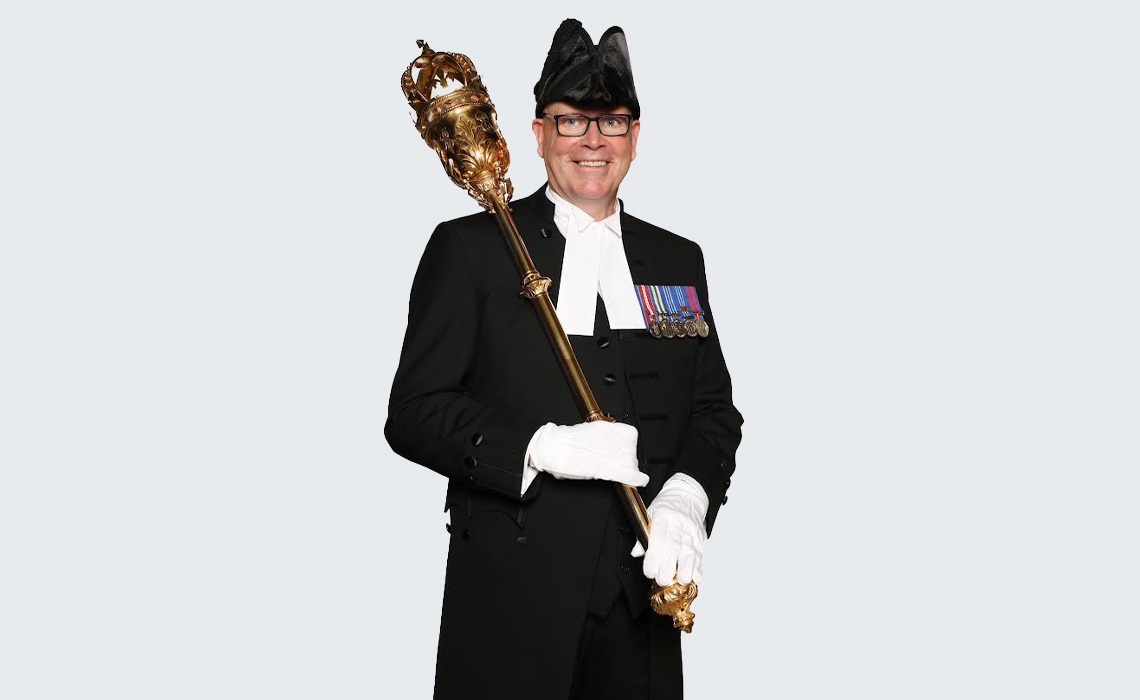This color photograph features a middle-aged man, likely of some royal or formal standing, captured against a white background. He is dressed in a distinguished black suit consisting of a long top coat, a black tuxedo jacket and pants, and a black vest over a white collared shirt with an expansive white lapel. His accessories include a white tie and immaculate white gloves. On his left lapel, five medals are prominently displayed. He holds an intricately carved golden scepter, the top of which is as large as his head, in his right hand. This man wears square-framed black glasses and is smiling, revealing his top row of teeth, while looking slightly off to the left. A unique decorative fabric hat with a fur-like texture and two black ear-like extensions rests on his head, contributing to his overall regal and ceremonial appearance.